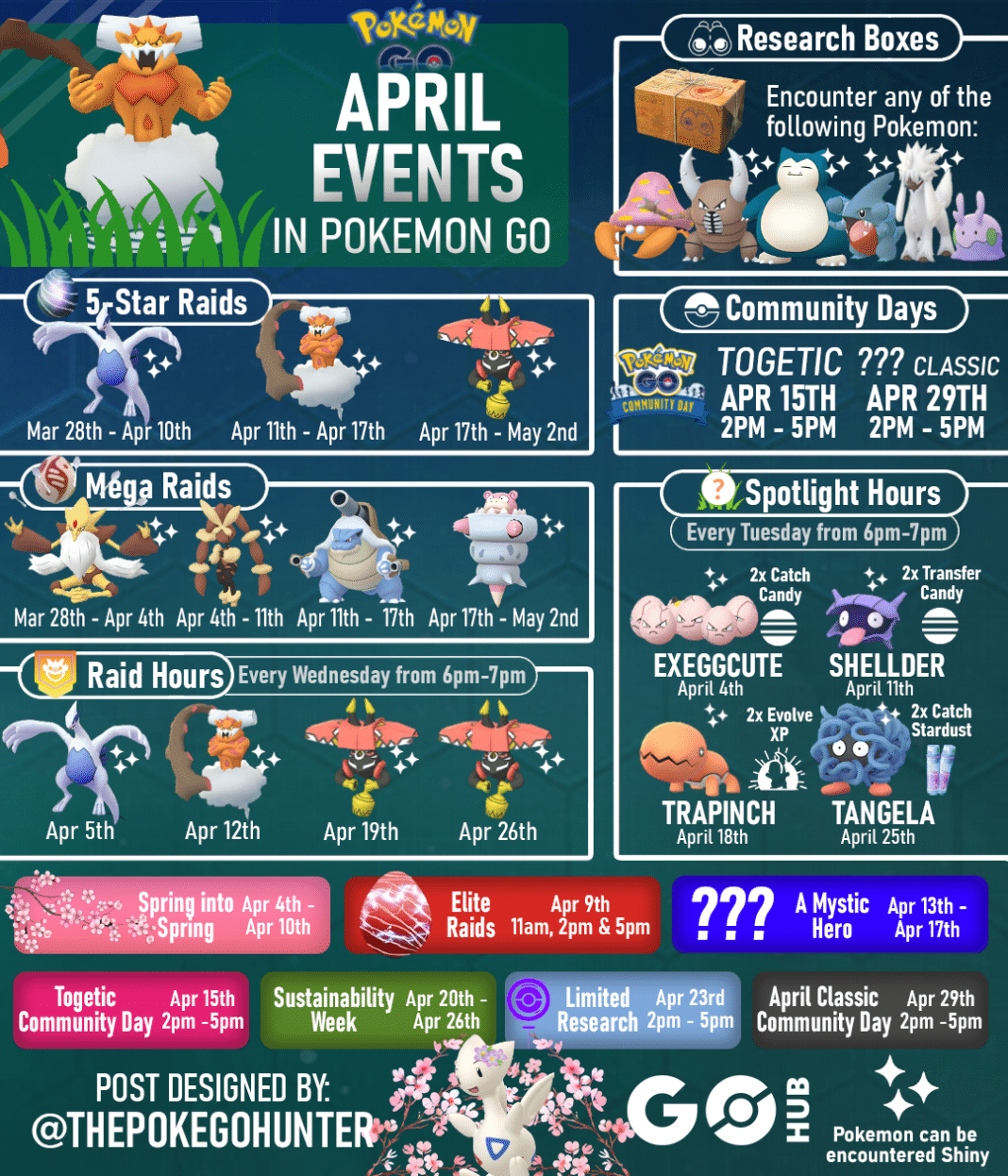The image features a detailed schedule of the April events for Pokémon GO against a blue background. The header includes "Pokémon April Events" prominently, indicating various activities and encounters for the month.

- **Research Boxes**: Players can expect encounters with various Pokémon.
- **Community Days**: Scheduled for April 15th and April 29th, from 2 p.m. to 5 p.m. These events offer special opportunities to catch featured Pokémon.
- **Five-Star Raids**: Available from March 28th to April 28th, with highlighted dates on April 11th and April 17th.
- **Mega Raids**: Divided into four intervals:
  - March 28th to April 4th
  - April 4th to April 11th
  - April 11th to April 17th
  - April 17th to May 2nd
- **Raid Hours**: Held every Wednesday from 6 p.m. to 7 p.m., on April 5th, April 12th, April 19th, and April 26th.
- **Spotlight Hours**: Occurring every Tuesday from 6 p.m. to 7 p.m., featuring:
  - Exeggcute with 2x catch candy on April 4th
  - Shellder on April 11th

This comprehensive schedule provides Pokémon GO players with various events to participate in throughout the month of April.